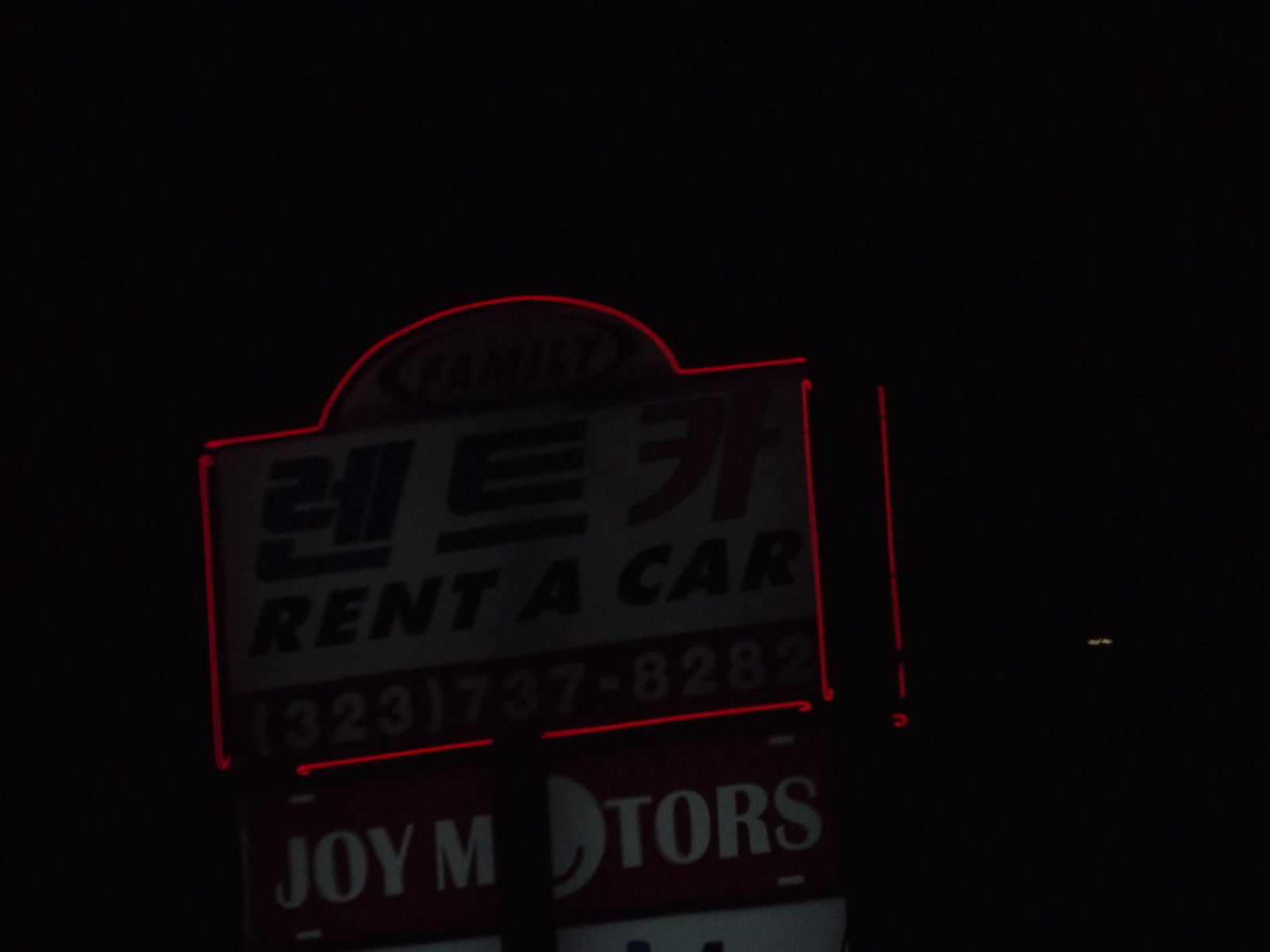This rectangular image, oriented horizontally, captures the deep hues of night with a stark black backdrop that accentuates the focal point of the scene: an illuminated sign. The sign is outlined by vibrant red neon lights, which provide the only light source, casting a faint glow but leaving the majority of the sign in shadow. 

At the top, there is an inscription, potentially in Chinese or Japanese characters, followed by the text "Rent a Car" in prominent black lettering against a white background. Directly beneath this, a phone number is boldly displayed: 323-737-8282. The lowest segment of the sign reads "Joy Motors," where the letter "O" in "Motors" is creatively depicted as a wheel, suggesting motion or automotive symbolism. The composition of the image combines elements of urban signage with a minimalist color palette, making the information stand out starkly against the enveloping night.